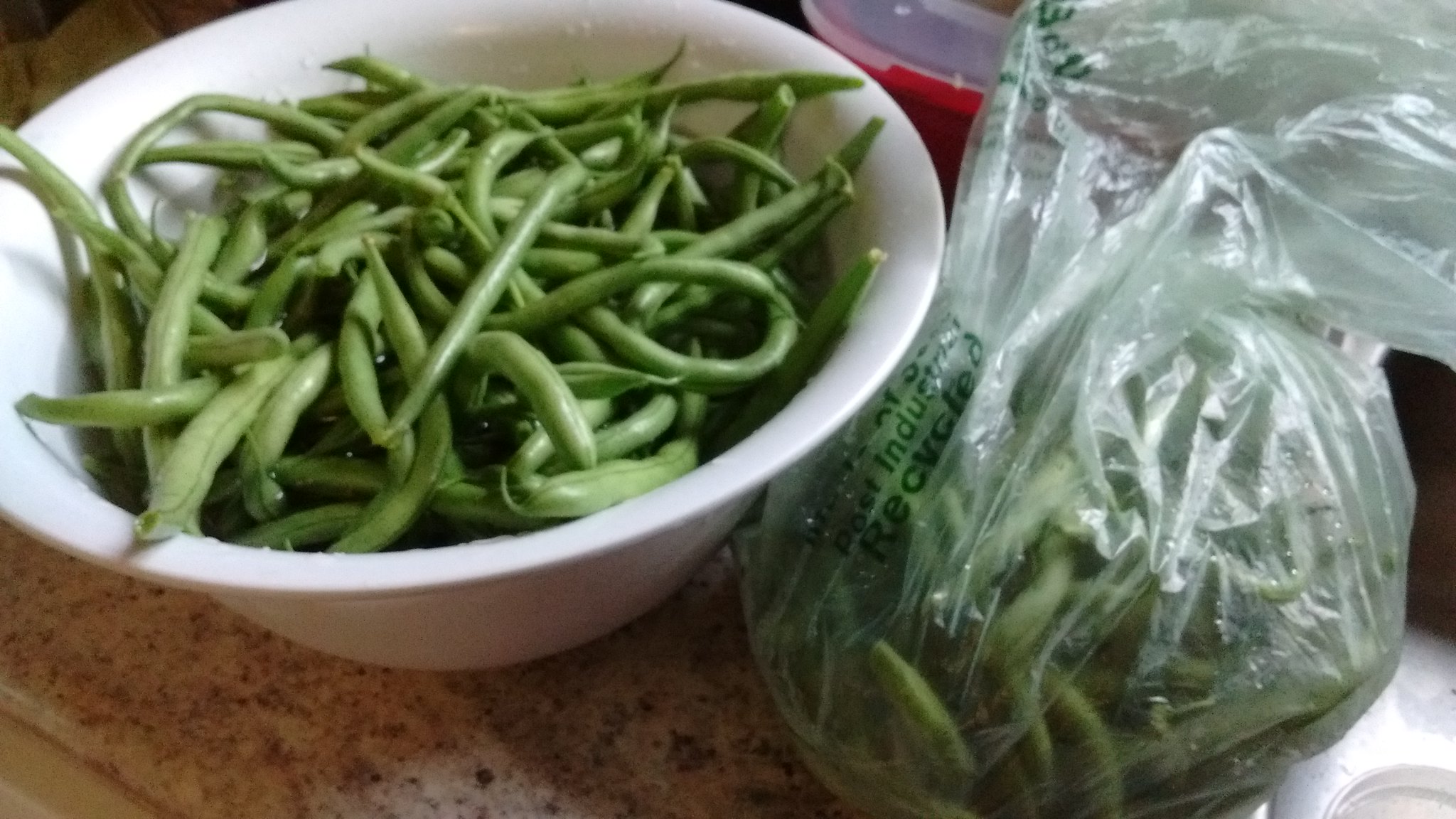This detailed photograph captures a close-up of a white porcelain bowl filled to the brim with long, shiny green beans, complete with their strings intact. The green beans are uncut and arranged in an overlapping, somewhat messy manner, giving a sense of abundance as they nearly spill over the sides of the bowl. To the right of this bowl sits a clear plastic grocery bag, potentially repurposed for harvesting or carrying the green beans, which appears to be similarly filled with more green beans. The bag has some green lettering on it, likely reading "recycle." Both the bowl and the bag rest on a tan granite countertop speckled with black, adding texture to the image, which is illuminated by a light source above, casting reflections on the glossy surfaces. Adding to the scene, a red container with a white lid, reminiscent of Tupperware, is visible in the background, hinting at further preparation or storage of food. The setting implies a harvest or preparation stage for a meal featuring these fresh green beans.